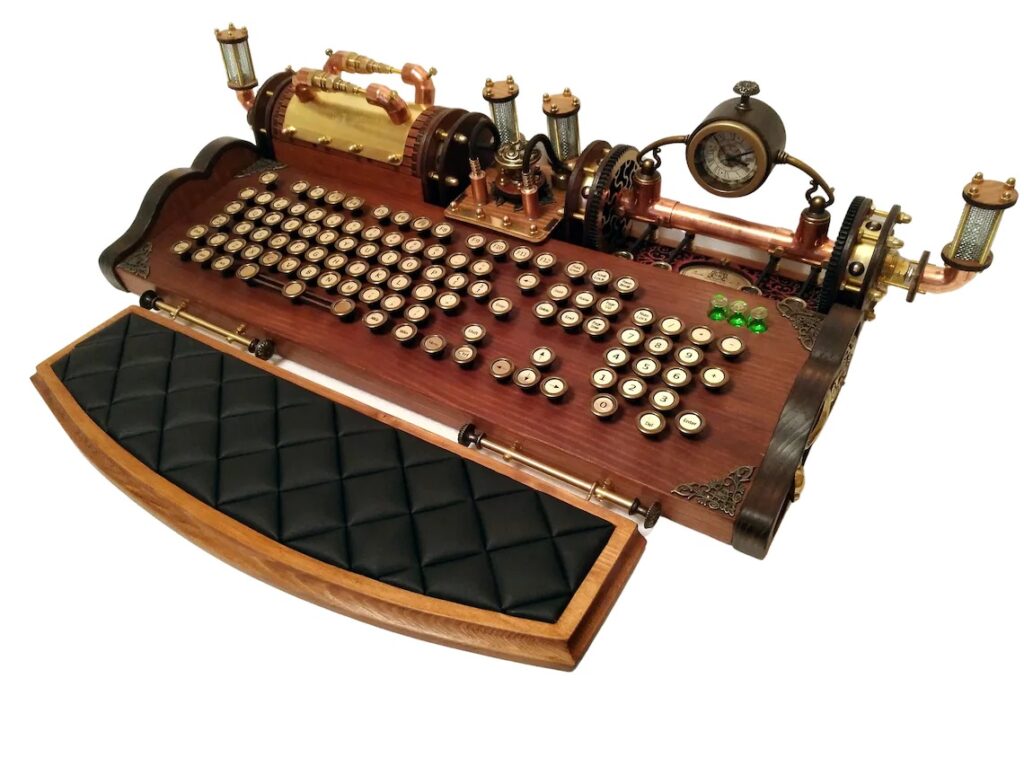Against a white background, the image showcases a meticulously designed, steampunk-inspired typewriter keyboard. The rectangular keyboard, approximately a foot and a half in length, features a dark brown wooden base with an array of off-white keys, each accented with a metal border, reminiscent of old typewriter buttons that require a firm press. The keyboard retains a modern layout, seamlessly blending antique aesthetics with contemporary design.

At the top of the keyboard, there is a series of intricate gold and brown gears, small cylinders secured with screws, and several valves, contributing to its steampunk motif. A prominent round dial resembling a clock or speedometer enhances this theme. Adding to the unique design, three little green gemstone-like embellishments are located in the upper right corner.

In front of the keyboard is an ergonomically designed wrist pad, which is slightly curved on one side and covered with a sleek black padding, ensuring both functionality and comfort. This pad, along with the other steampunk elements and valves adorned with glass tubes that might contain lights, solidifies the keyboard's fusion of antique charm and modern innovation.